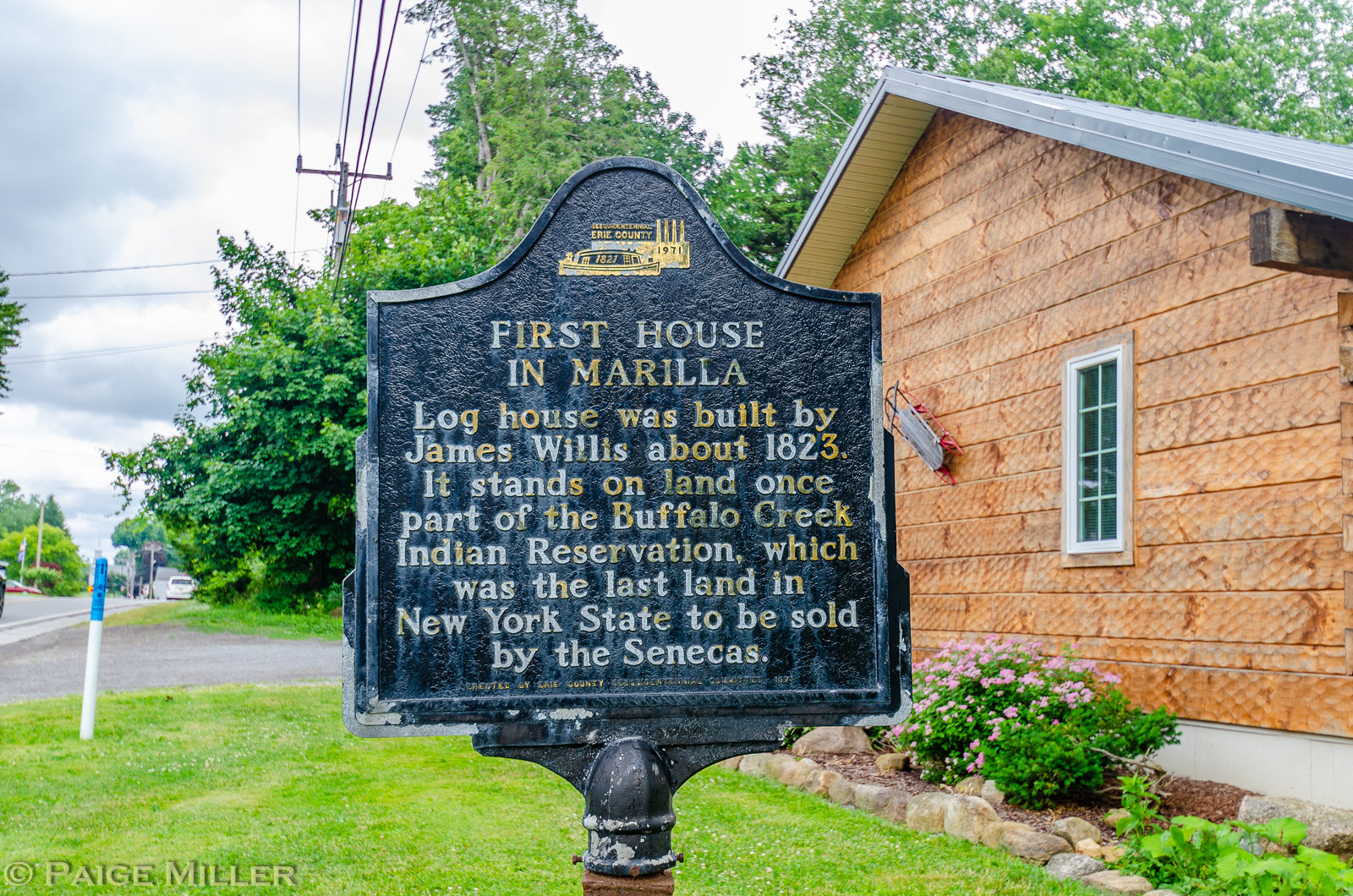The image depicts a historic scene featuring a detailed sign and a wooden cabin. The sign, which is black with gold lettering and likely made of a hard material such as stone or bronze, is mounted on a metallic pole. It reads: "First house in Marilla. Log house was built by James Willis about 1823. It stands on land once part of the Buffalo Creek Indian Reservation, which was the last land in New York State to be sold by the Senecas." The sign also contains a logo at the top, which includes the text "St. Quince, St. Daniel, Erie County, 1971-1821," and a depiction of a train or boat.

On the right side of the sign stands an old wooden cabin featuring planked exterior walls, a triangular grey roof, and a small window. Flowers with pink petals and green leaves are neatly planted at the base of the cabin, surrounded by rocks. To the left of the sign, there is a grassy area with another post nearby. 

In the background, tall trees stretch upwards towards a sky filled with white and grey clouds, with power lines running across the scene. There’s a road behind the house, with cars visible, adding to the sense of an active environment. The foreground includes a neat grassy lawn, which is accented by some scattered flower bushes. A watermark in the bottom left corner states "Copyright Page Miller."